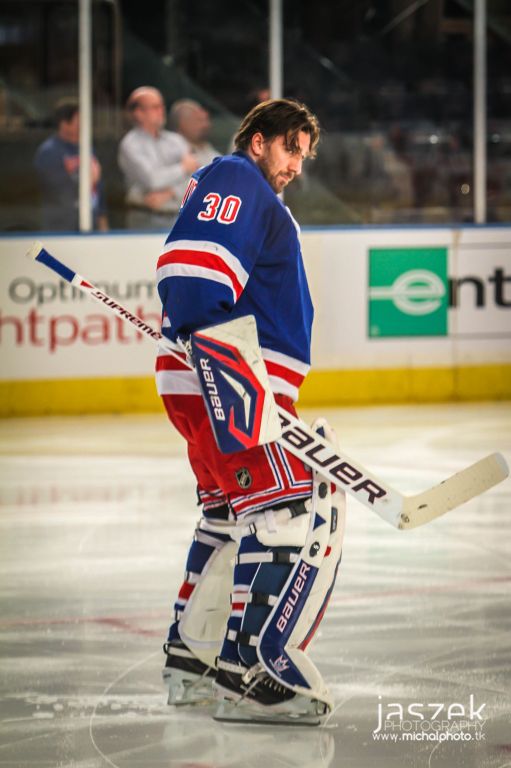In this detailed photograph, we see a solemn-faced Caucasian man on a hockey rink, captured from the side. The man, a goalie, is dressed in full gear, including heavy pads and a distinct hockey uniform. He sports black ice skates with silver blades, white bottoms, and large white leg pads with blue sides, featuring the "Bauer" logo in white font. His white leg straps are secured with black buckles, complementing his blue, red, and white striped leggings. He is wearing red shorts with white stripes and a blue jersey adorned with red and white stripes on the sleeves. The jersey prominently displays the number 30 outlined in white. The goalie holds a large white hockey stick in his right hand and has medium-length brown hair and a scruffy beard, hinting at a man in his 30s or 40s. Notably, he isn’t wearing a helmet, likely indicating a break or warm-up session. The photograph reveals a mostly empty background with few spectators and the rink's protective glass visible. A watermark reading "Jasek Photography" with the website "www.michalphoto.tk" is in the lower right-hand corner. The man's intense gaze and serious demeanor add to the depth of this compelling sports image.